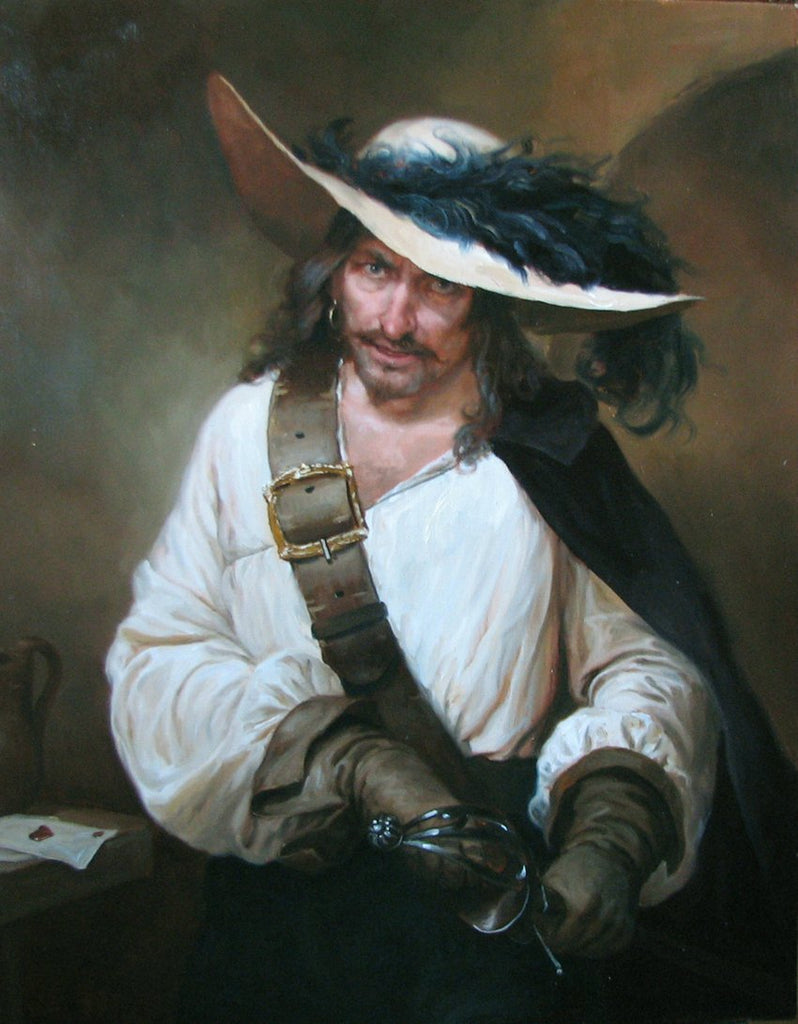A painting or digital illustration depicts a man dressed in attire suggestive of a pirate, buccaneer, or Spanish conquistador, set against a brown, cave-like backdrop. The central figure is a weathered individual with a bold nose and light skin, staring directly at the viewer. His long, curly hair is brown with hints of gray, cascading to his shoulders. He sports a short, pointy mustache, some stubble on his chin, and an earring in his left ear. He wears a flamboyant white hat adorned with a plume of blue and black feathers draping down the side, tilted slightly down and to the right. His apparel includes a baggy, white puffy shirt, long brown gloves, and a wide brown belt that stretches diagonally from his shoulder to his waist, securing a black cape over his left shoulder. The man's right hand grips the base of a silver-handled rapier, with its blade extending down towards the bottom right of the image, while his left hand holds the sword's base. The scene includes a wooden table at the lower left, featuring a white playing card with a heart in its center and the partial view of a mug with a handle pointing rightwards. Additionally, there appears to be some sort of letter with wax on it nearby. The overall scene is rich with detail, capturing the essence of the character and the setting.